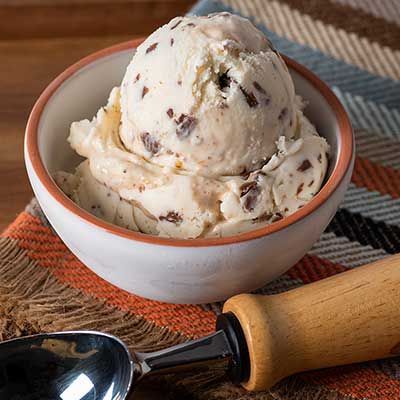The overhead photograph captures a white bowl with a trim of orangish-red or camel color on the lip, situated on the lower left edge of a striped placemat. The placemat features diagonal stripes of various colors, including orange, brown, bluish-gray, white, cream, and green, with some stripes being solid and others patterned. Inside the bowl are several generous scoops of vanilla ice cream, adorned with black and brown speckles that may suggest the inclusion of nuts or chocolate chips. In the foreground, below the bowl, lies a metal ice cream scooper with a wooden handle, positioned ready for use. The placemat covers almost the entire scene, while a small portion of the table is visible in the upper left corner.